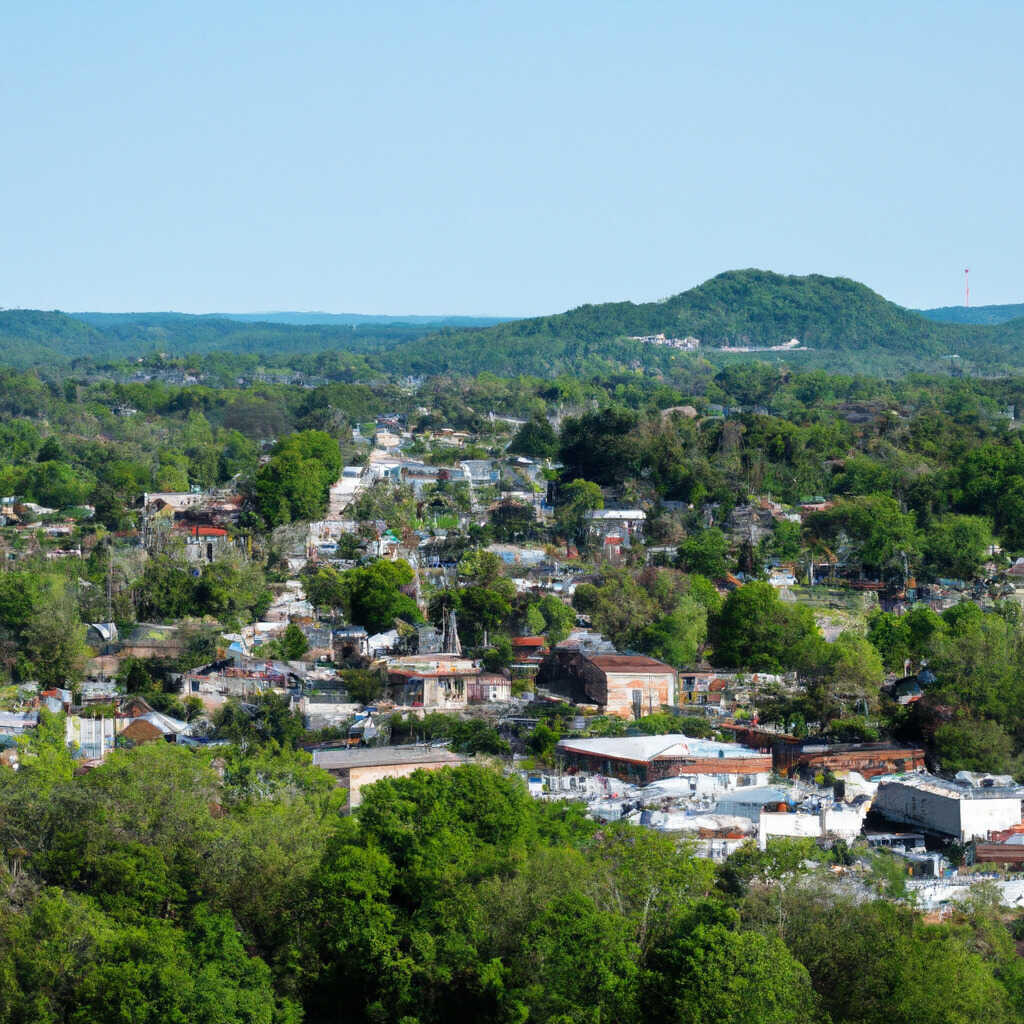This aerial photograph, likely taken from an elevated vantage point such as a hill or mountain, showcases a small town nestled within a lush, green landscape. The town, comprising about 40 buildings, features white and brown structures no taller than four stories, interspersed with a dense array of trees. The foreground of the image displays a rich tapestry of trees and bushes, continuing a pattern of alternating buildings and trees throughout the scene. In the distance, a scenic backdrop of low mountain ranges adds depth to the composition, with another separate town visible on the hills. The sky above is a clear, vibrant blue, suggesting a warm climate, possibly indicative of a region like South America. The overall impression is of a quaint, seemingly third-world village enveloped by natural greenery against the striking blue sky, presenting a harmonious blend of nature and human habitation.